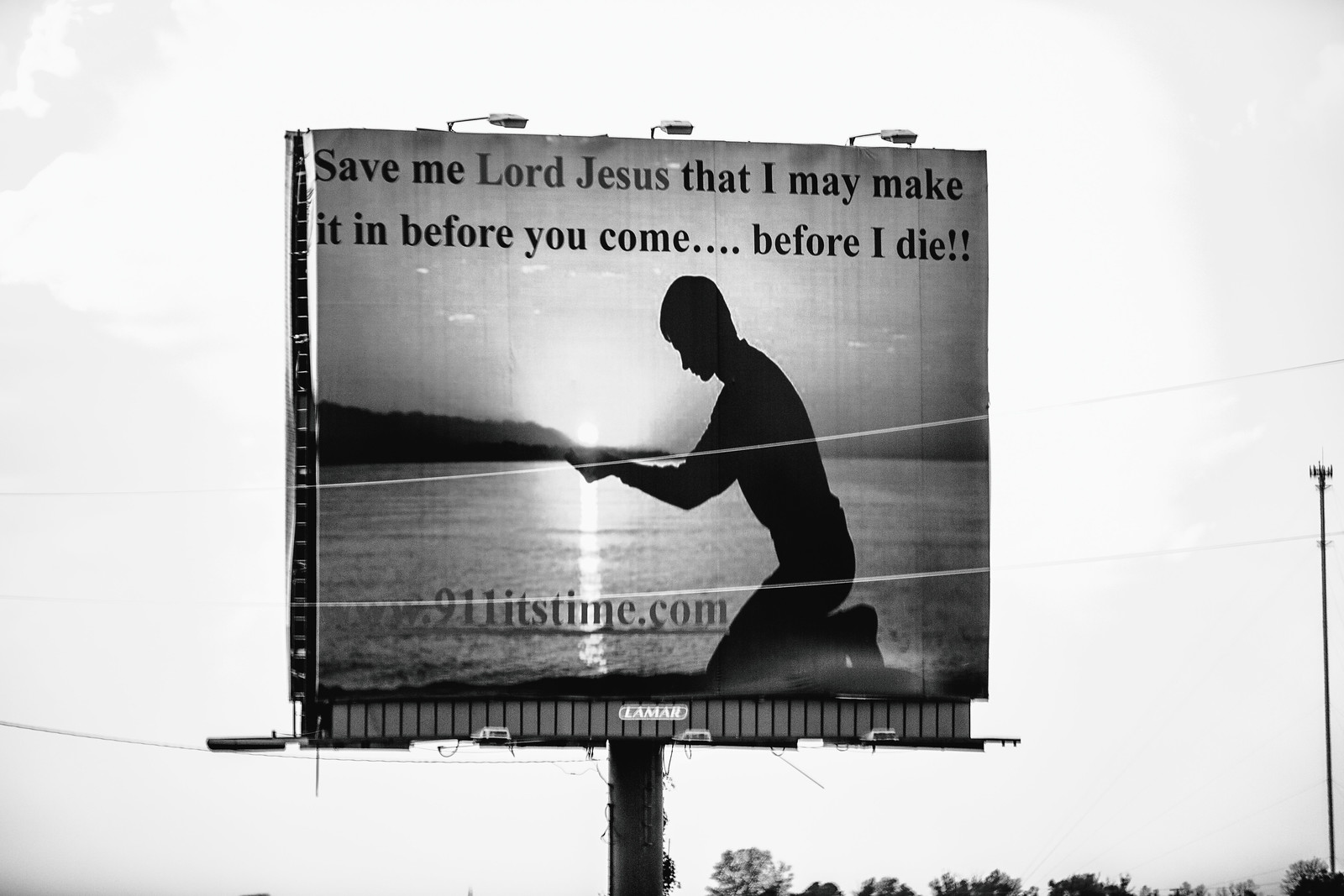In this striking black and white image, the focal point is a towering billboard set against the backdrop of a sky punctuated by a distant tree line, a light pole, and a network of electrical wires. Dominating the billboard is a powerful illustration of a man kneeling by a vast body of water—possibly an ocean or lake—his hands cupped as if cradling the sun. The poignant quote on the billboard reads, "Save me, Lord Jesus, that I may make it in before you come, before I die." Below this haunting plea, the website www.911itstime.com is prominently displayed. The contrasting elements and the emotional weight of the message combine to create a deeply evocative scene.